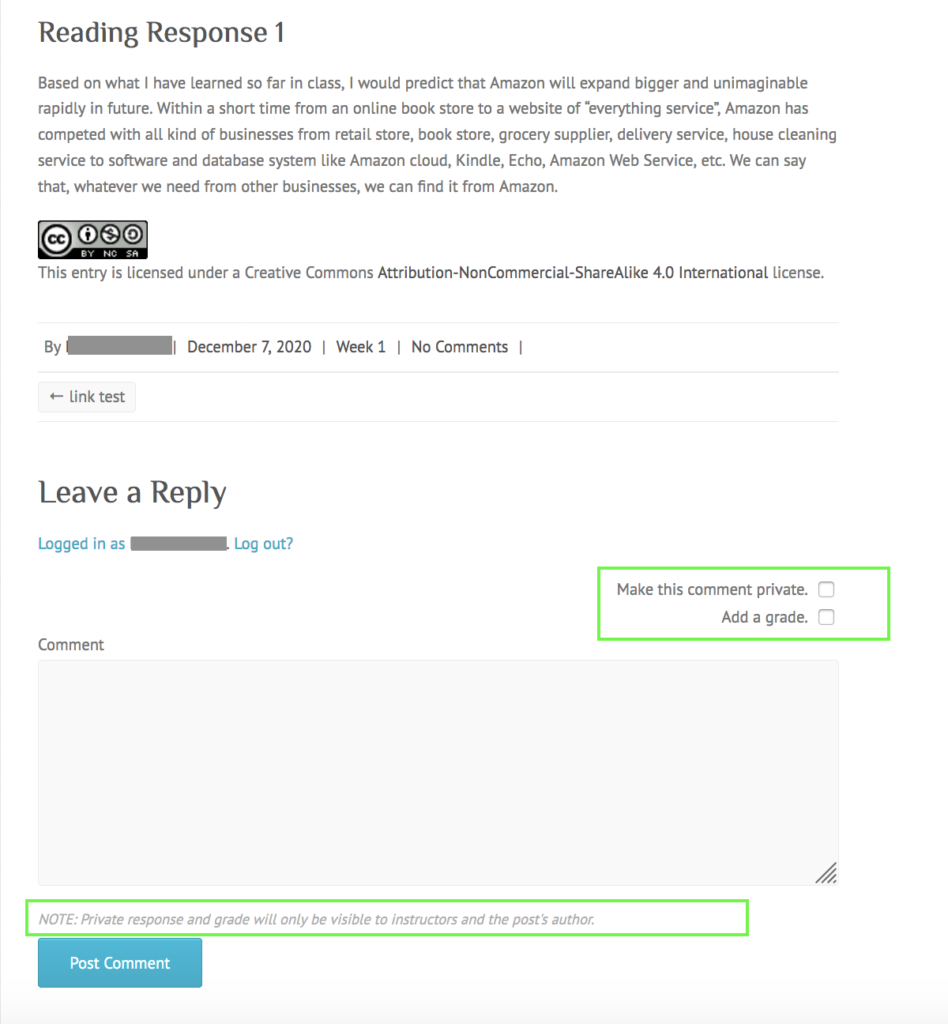**Descriptive Caption:**

The image displays an annotated screenshot of an online academic discussion platform titled "Reading Response 1." At the top, the student writes a predictive analysis regarding Amazon's future growth: "Based on what I have learned so far in class, I would predict that Amazon will expand bigger and unimaginable rapidly in the future. Within a short time, from an online bookstore to a website of everything service, Amazon has competed with all kinds of businesses from retail store, bookstore, grocery supplier, delivery service, house cleaning service, to software and database system like Amazon Cloud, Kindle, Echo, Amazon Web Service, etc. We can say that whatever we need from other businesses, we can find it from Amazon." 

Below this text is a Creative Commons license indicating that the entry is licensed under a Creative Commons attribution-noncommercial-sharealike 4.0 international license. The author's name is obscured by gray marker-like text, denoted as "by blank." The post is dated "Published on December 7, 2020, week one, no comments." To the right, a small button labeled "Link Test" with a left-pointing arrow is present.

Underneath this section, the interface includes options such as "Leave a Reply" with the name of the logged-in user obscured again, followed by "Log out, question mark."

Annotations in bright green highlight specific areas for further action or comments. The text "Make this comment private" is enclosed within a green rectangle, suggesting a checkbox feature to control the privacy of the student's response. Another green box encircles the note: "Note, private response and grade will only be visible to instructors and the post's author." Following this is a blank comment box and a "Post Comment" button.